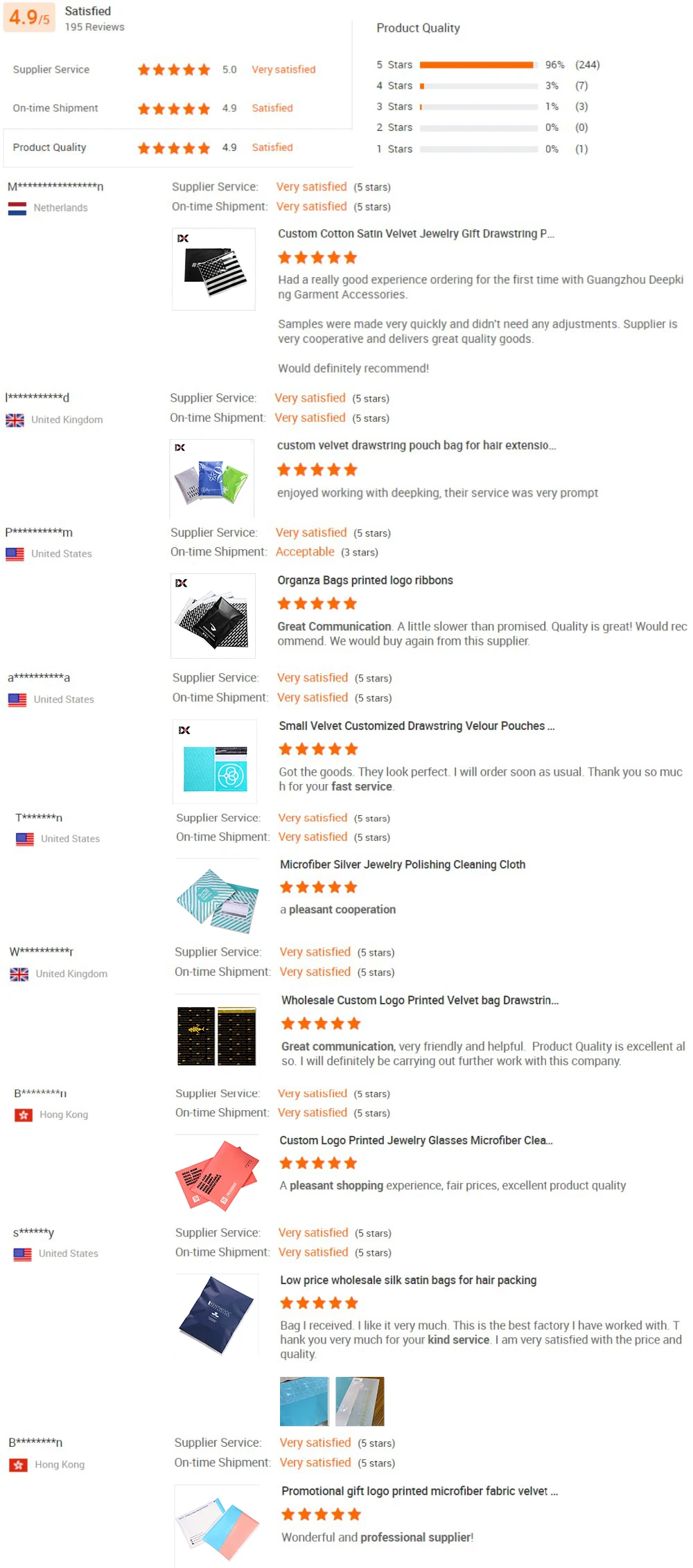This image is a blurry screenshot of a product page resembling an Amazon-like website. The layout displays various customer reviews for a specific seller, with each review including the reviewer's name at the left. The reviews detail what the customers bought, accompanied by the ratings they gave, which are mostly five stars out of five. Some reviews also include customer-uploaded images of the received products, showcasing personal experiences beyond the standard product images. At the top of the image, there is a summary of the seller’s performance, indicating that over 90% of the reviews are five-star ratings, with a small percentage being four stars. No three, two, or one-star reviews are visible, as indicated by the absence of orange bars in those sections. Despite the small text making it difficult to read specific comments, the overall impression is of a highly-rated seller with predominantly positive feedback.